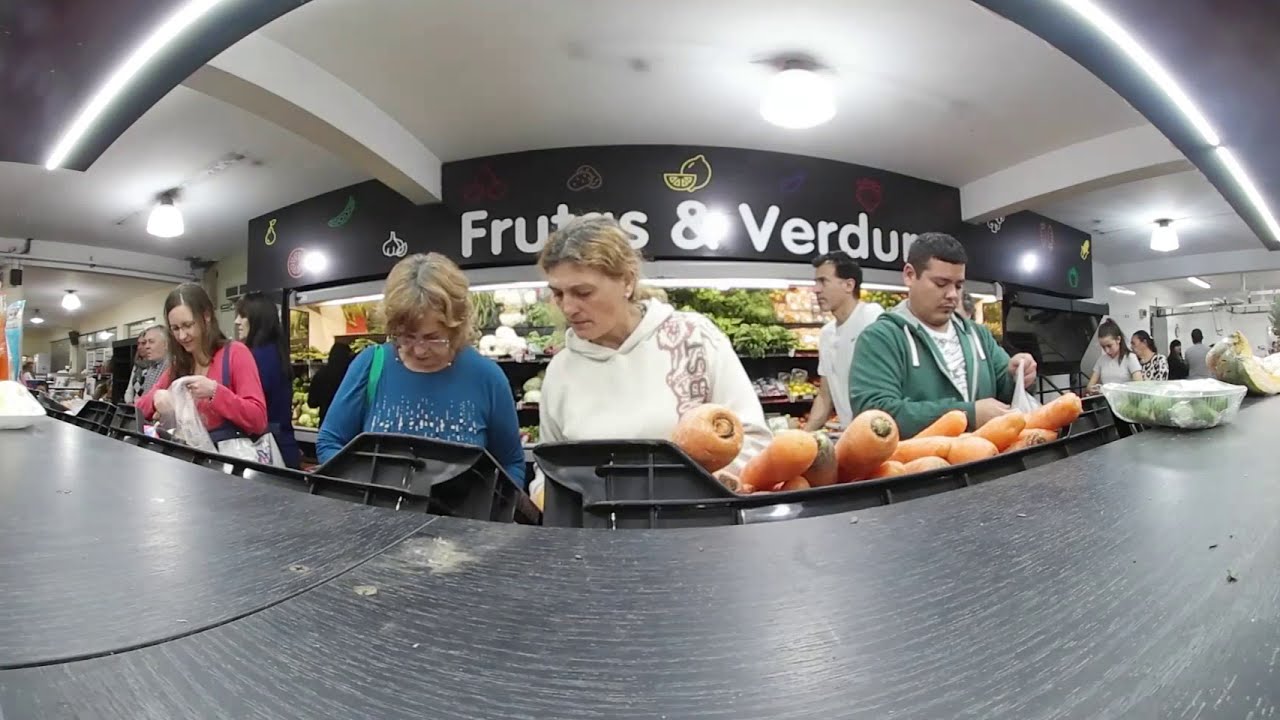The image depicts a bustling indoor produce section of a grocery store captured using a panoramic lens, which creates a curved effect around the edges, making the area appear more condensed than it actually is. Numerous people are engaged in selecting fresh vegetables from large black plastic bins prominently positioned at the forefront. The most striking produce in these bins are the vibrant orange carrots on the right. 

The scene is vividly lit by both fluorescent light strips and round ceiling lights set against a white ceiling with white support beams. Directly in front of the camera, placed atop a black wooden counter, multiple individuals are engrossed in their shopping. Notable among them are a woman in a white sweater with blonde hair, who is looking down at something another blonde woman with glasses in a blue top is pointing out. To their left stands another woman, and to their right, a man in a green zip-up sweater stands next to a man in a white polo shirt. 

In the background, other shoppers are dispersed along the aisles, some walking, while others are further down, filling their bags with produce. The opposite display counter, also loaded with vegetables, features cartoon illustrations of fruits and vegetables along with partially obscured text, spelling out "FRUITS & VERD..." The left side of the image appears to lead toward the checkout area. Overall, the space, though not very large, is clearly bustling with activity under the bright, well-distributed lighting.